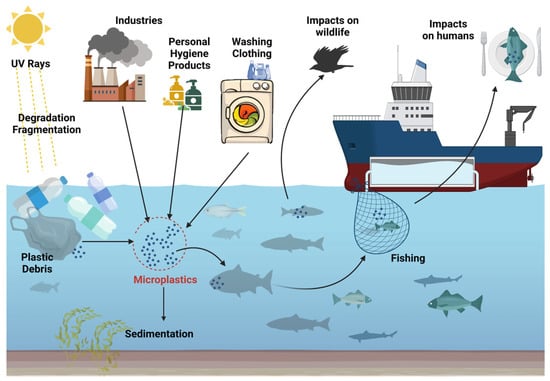The diagram illustrates the multifaceted impact of fishing on humans and wildlife through a comprehensive, detailed cross-section of the ocean. In the underwater portion of the image, blue water contains various fish and plastic debris identified to the far left, labeled as "plastic debris" in black lettering. An arrow from this debris points right to a dotted circle filled with blue dots, captioned "microplastics" in red, indicating how plastics break down in the water. Another arrow from the circle points downwards to the seabed, labeled "sediment," highlighting the accumulation of microplastics in the ocean floor. To the right within the water, fish are shown, with an arrow from a fish's tail leading upwards into a fishnet, representing their capture. Continuing upwards, another arrow leads right to a dinner plate with a fork and knife beside a fish, labeled "impact on humans."

Above water, the diagram depicts several contributing factors. In the top left corner, the Sun emits UV rays toward plastic debris, labeled "degradation, fragmentation," signifying the breakdown of plastics into microplastics. An adjacent industrial building labeled "industries" implies pollution sources. To the right, two bottles, one gold and one green, represent "personal hygiene products," with arrows pointing down to the microplastics. Further right, a washing machine illustrates "washing clothing" with similarly directed arrows toward the microplastics. Center-right, an all-black outline of a bird points to "impacts on wildlife," emphasizing ecological consequences. Lastly, on the top right, a blue and red fishing boat with a white captain's fuselage is depicted on the water's surface, completing the depiction of the fishing process and its broad-reaching impacts.